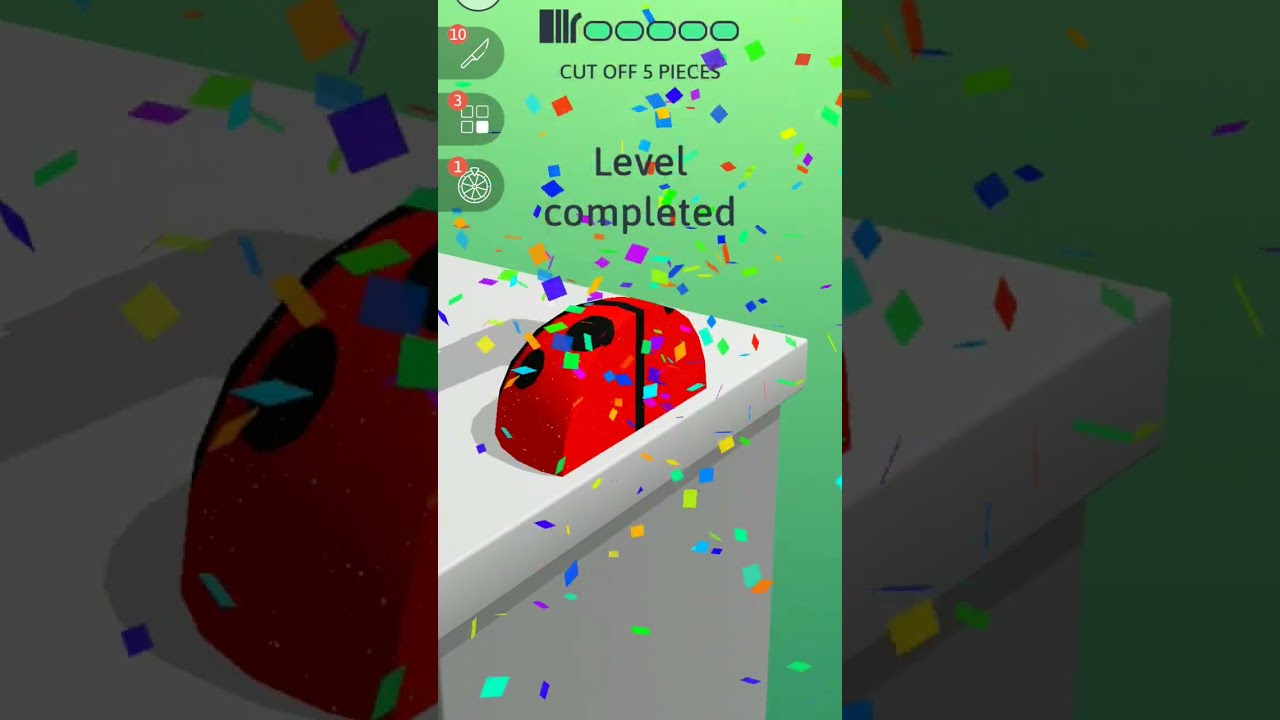The image depicts a computer-generated scene, likely a screenshot from a mobile game, featuring a white tabletop in the bottom left corner set against a green wall. Central to the image is a red, quarter-spear-shaped object adorned with two large black dots near its top and a prominent black line dividing it in the middle. Confetti in various vibrant colors, including gray, green, light blue, dark blue, purple, green, orange, and yellow, cascades from the ceiling, adding a festive atmosphere. Text overlays the image with "level completed" in green letters positioned on top, while the instruction "cut off five pieces" is centered above five small green circles at the top middle of the screen. This scene encapsulates a moment of triumph, filled with colorful celebration and clear objectives in a gaming context.